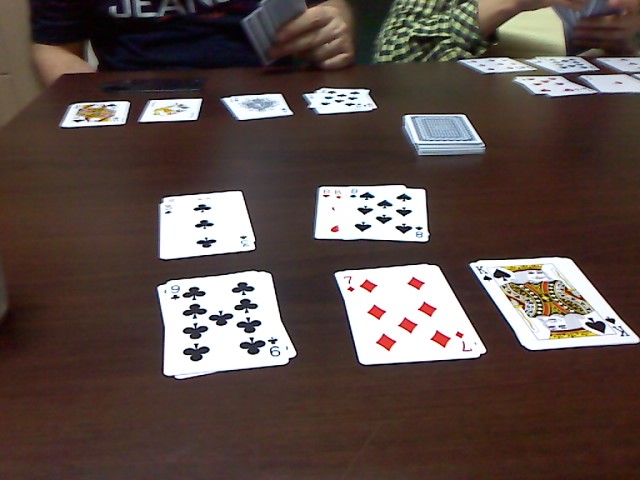In this photograph, a dark brown, glossy wooden table dominates the scene. Spread across the surface are multiple piles of cards, including a noticeable pile of nine cards at the top, a pile of seven cards, and one featuring a King. Toward the upper part of the image, partially visible behind the table, are at least two individuals with light skin tones. On the left, one person is dressed in a navy t-shirt adorned with white text, possibly spelling out "jeans" given the visible bottom half of the letters J-E-A-N. On the right, the second individual sports a green and yellow or white checkered long-sleeve shirt. Only parts of their arms and one hand are discernible, adding a human element to the focused arrangement of the playing cards.